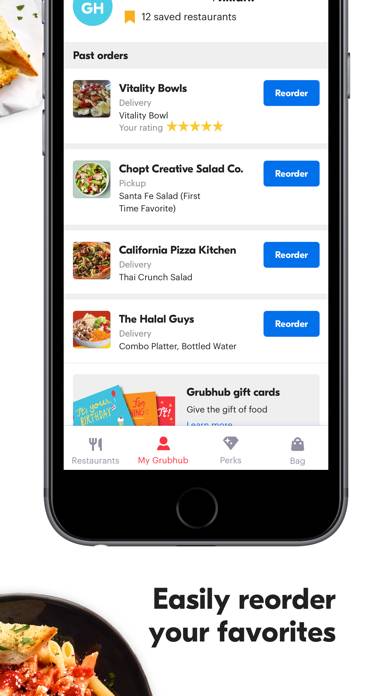This digital web poster features a black-framed iPhone at its center, showcasing a specific app on its screen. The phone displays a user-friendly interface with a white background, where various restaurant listings are arranged horizontally. Each listing includes a blue "Reorder" button situated on the right side. From top to bottom, the restaurant listings are as follows:

1. Vitality Bowls: Accompanied by a square image of a food bowl on the left, the listing indicates "Vitality Bowls" in black text, with the word "delivery" in gray, and a five-star rating below.
2. Chopped Creative Salad Co.: Featuring an image of a salad bowl, this listing shows "Chopped Creative Salad Co." in black text, "pick-up" in gray, and "Santa Fe Salad" beneath.
3. California Pizza Kitchen: Highlighted by a picture of a pizza, this listing reads "California Pizza Kitchen" in black text, with "delivery" and "Thai Crunch Salad" mentioned below.
4. The Halal Guys: Displaying an image of a combo platter, the listing indicates "The Halal Guys" in black text, "delivery," and "Combo Platter, bottled water" beneath.

Beneath the phone image, a black text caption reads, "Easily Reorder Your Favorites," emphasizing the app's convenience. The bottom left corner of the poster subtly features a black plate of pasta, partially visible and adding a culinary touch to the overall composition.